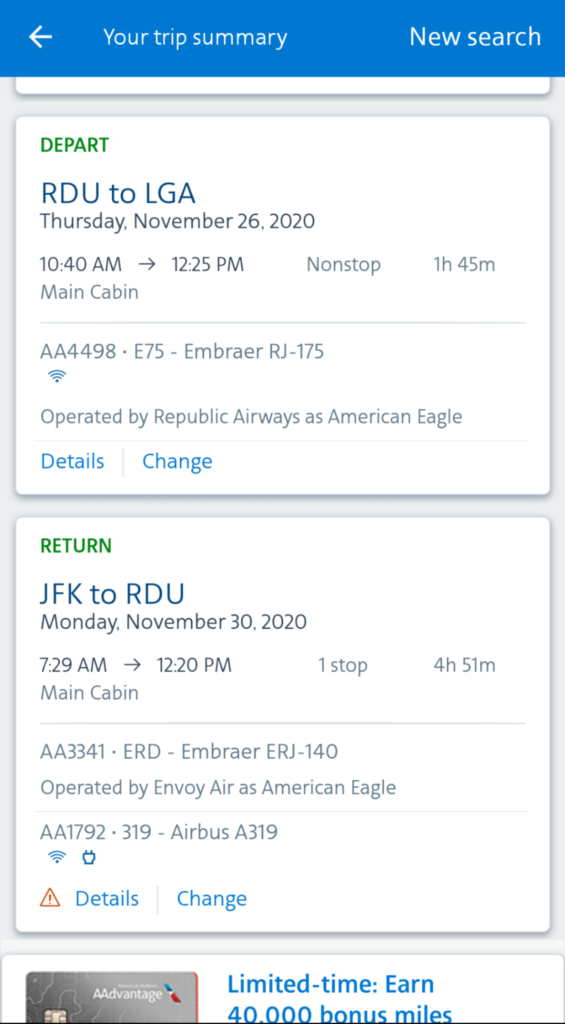This image is a screenshot from a mobile device displaying flight information. At the top, there's a blue bar with a white back arrow on the left, and the text "Your Trip Summary" in the middle. On the upper right corner, it says "New Search." Below this, there are two white blocks of information. 

The first block details the departure flight with green text: "Depart: RDU to LGA, Thursday, November 26, 2020, 10:40 a.m. to 12:25 p.m., non-stop, 1 hour 45 minutes." Below this information, there are options to view details and change the flight.

The second block outlines the return flight: "Return: JFK to RDU, Monday, November 30, 2020, 7:29 a.m. to 12:20 p.m., one stop, 4 hours 51 minutes." Similarly, there are options to view details and change the return flight.

At the bottom of the screenshot, a portion of an American Airlines AAdvantage card is visible.